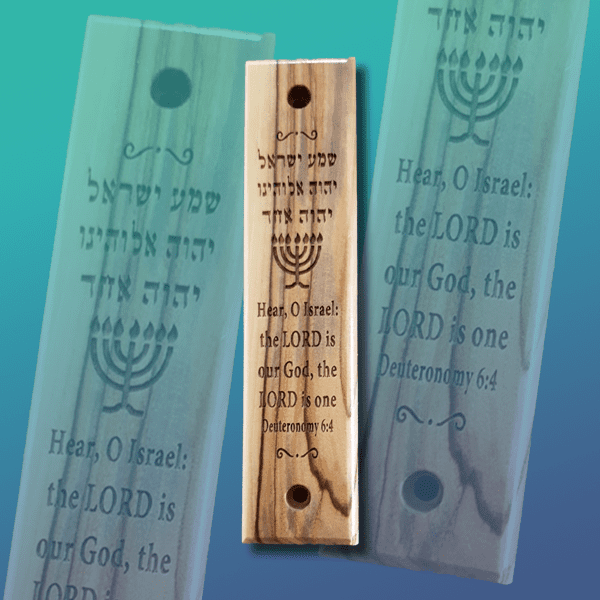The artwork depicts a central piece of wood bearing religious inscriptions prominently displayed in the foreground against a blue background. This central piece is smaller but more detailed in its presentation. It features an oval hole at the top and another at the bottom, likely for attachment purposes. Below the top hole, there is an ornamental design resembling an inverted mustache with a dot in the middle. The main inscription on the wood is in Hebrew, followed by a menorah, and then an English translation from Deuteronomy 6:4, which reads: "Hear O Israel, the Lord is our God, the Lord is one." Below this text is the same ornamental mustache-like design and the bottom oval hole. 

In the background, two larger but faded versions of the same wooden piece are superimposed at an angle of about 30 degrees to the right. These echo the exact same design, words, and holes as the central piece, displaying a consistent wood grain pattern. The background coloration transitions from a greenish-teal at the upper left to a deep blue towards the bottom right, creating a radiating effect that emphasizes the central wood piece.